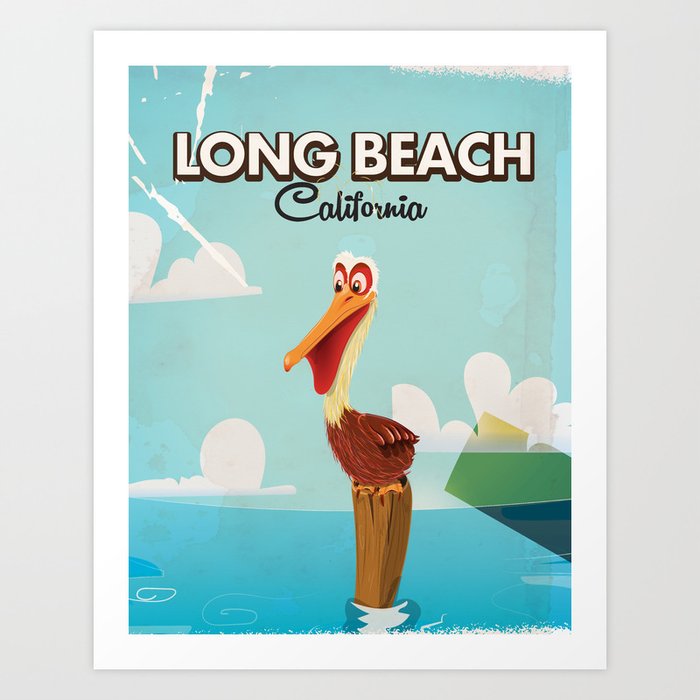This detailed color illustration, styled as wall art, is framed in white and set against a light gray background in portrait orientation. At the center of the image, a comical pelican is perched on a brown wooden post rising from the dark blue ocean. The pelican features a reddish-brown body, a cream-colored neck, and a white forehead. Its long yellow beak opens to reveal a red inner mouth. Red rings accentuate its eyes, which are raised for a humorous effect. 

Above the bird, white bold text with a black drop shadow spells out "LONG BEACH" in all caps, followed by the word "California" in a delicate black script font. The background of the image showcases a light blue sky filled with fluffy white clouds. To the right side, a multicolored rectangle adds a unique touch, displaying a landscape with a yellowish tint to the clouds, a greenish hue to the sky, and a darker blue tint to the water.